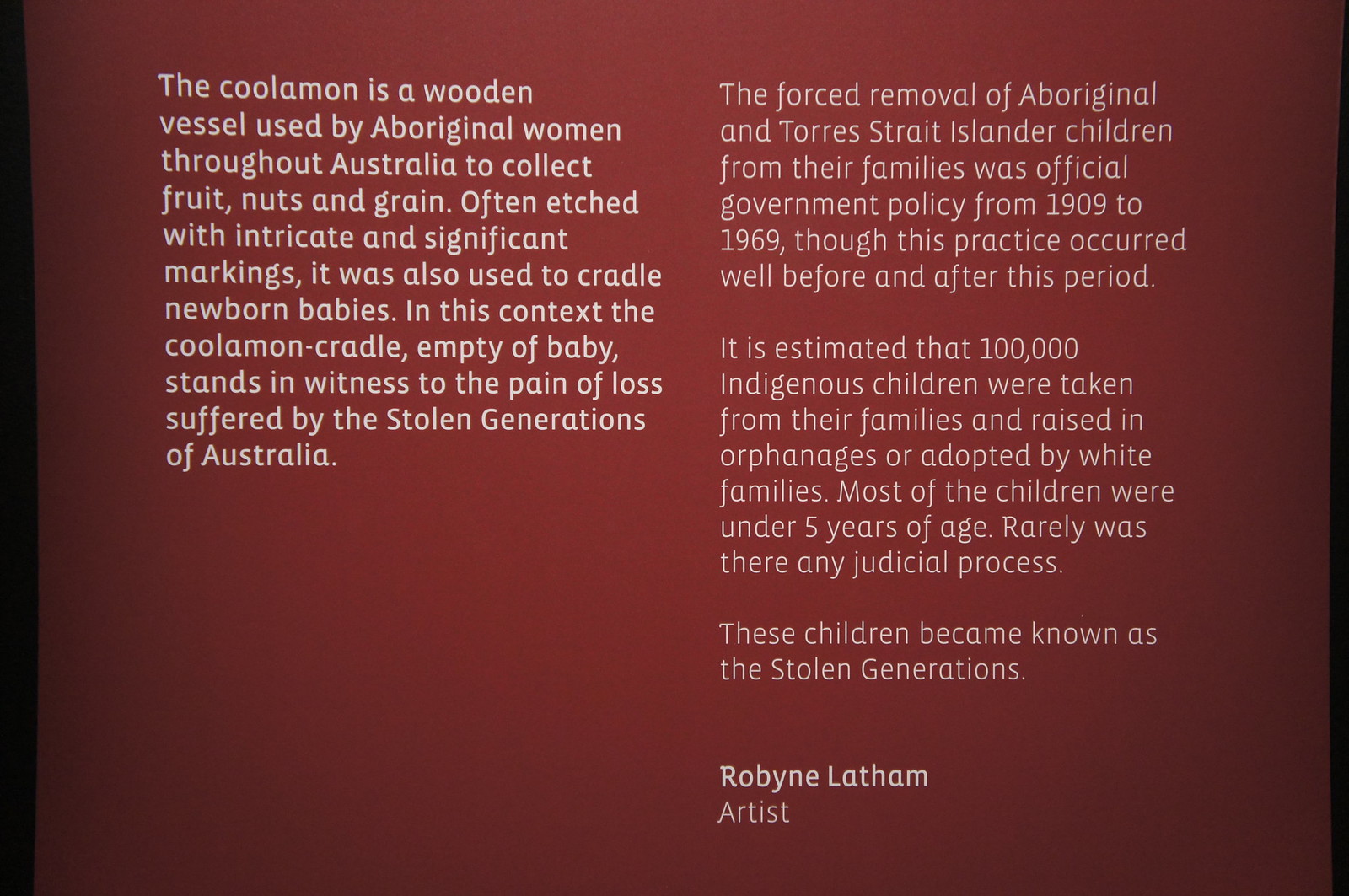The image features a brownish-red background with white print text displayed in two columns. The first column contains about ten sentences, while the second column has three short paragraphs. The text is an informative placard explaining that the Kulamon is a wooden vessel traditionally used by Aboriginal women in Australia to collect fruits, nuts, and grain. It was also often used to cradle newborn babies. The placard elaborates that in the context of the Stolen Generations—when an estimated 100,000 Indigenous children were forcibly removed from their families from 1909 to 1969, as part of official government policy—the empty Kulamon cradle symbolizes the collective pain and loss these communities suffered. This devastating practice saw children, mostly under five years of age, taken without judicial process and placed in orphanages or adopted by white families. The text is attributed to artist Robin Latham, who authored this poignant piece.